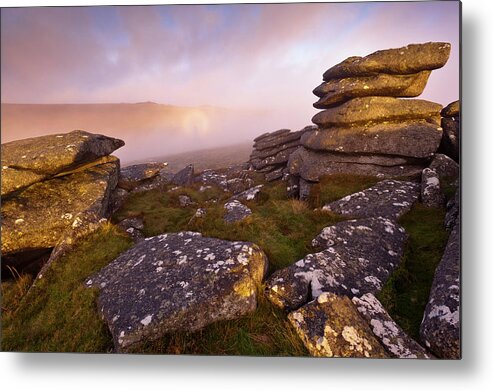This striking image captures a serene, rugged landscape featuring an array of flat, gray rocks with white speckles, some positioned singly while others are artfully balanced on each other. In the foreground, clusters of these rocks rest on a bed of lush grass, creating an inviting contrast. As the eye travels further back, the landscape appears more barren, dominated by stacked rocks leading to hazy, distant hills under a blue sky. The sky itself is a mesmerizing blend of purple, orange, red, and yellow hues, suggesting either a sunrise or sunset, with soft, pink-tinged clouds and a touch of fog enhancing the ethereal atmosphere. The sun casts a yellow reflection near the horizon, and the scene is framed by a black border, reminiscent of a photograph hanging on a white wall. Shadowing on the right side of this framed image hints at light coming from the top left, creating a play of light and shadow that adds depth to this mountain scenery.